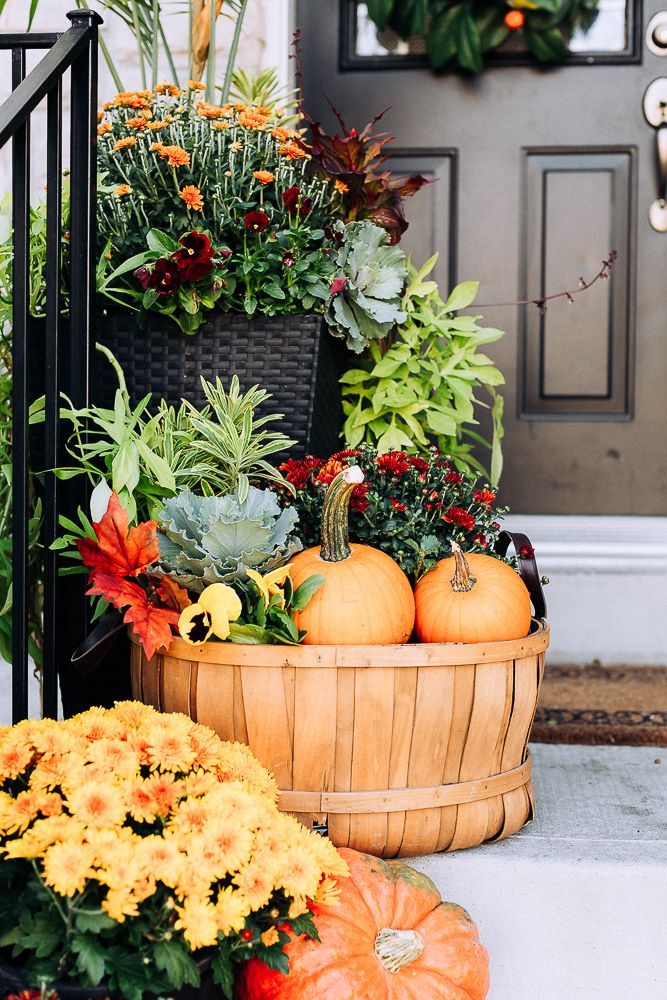This image, reminiscent of a scene from Better Homes and Gardens, captures a stunning, up-close view of a home's front porch steps in daytime. Dominating the left side of the image is a black cast iron railing, which elegantly complements the pristine white stairs. The focus is on the decorative elements adorning the steps, crafted into a harmonious autumn display.

On the bottom step, vibrant yellow mums with orange centers and lush green leaves spill out, setting a cheerful tone. Nestled among the blooms is a large pumpkin, distinguished by its orange hue with subtle green flecks. Just above this, the next step holds a natural wooden basket brimming with autumnal delights—two small pumpkins with elongated stems, surrounded by foliage in rich hues of oranges, dark reds, and varied greens.

The topmost step features a sophisticated black wicker basket overflowing with a medley of autumn flowers, predominantly in shades of vibrant orange. The multitude of smaller blooms creates a lush, full appearance.

Just beyond the steps, the dark brown front door becomes visible, adorned with a gold handle and partially obscured by an autumn wreath that hangs gracefully from the center. This wreath is hinted at by its ornate, season-appropriate décor, blending seamlessly with the overall autumnal theme of the porch.

This detailed and meticulously styled scene evokes a cozy, festive ambiance, perfect for the fall season.